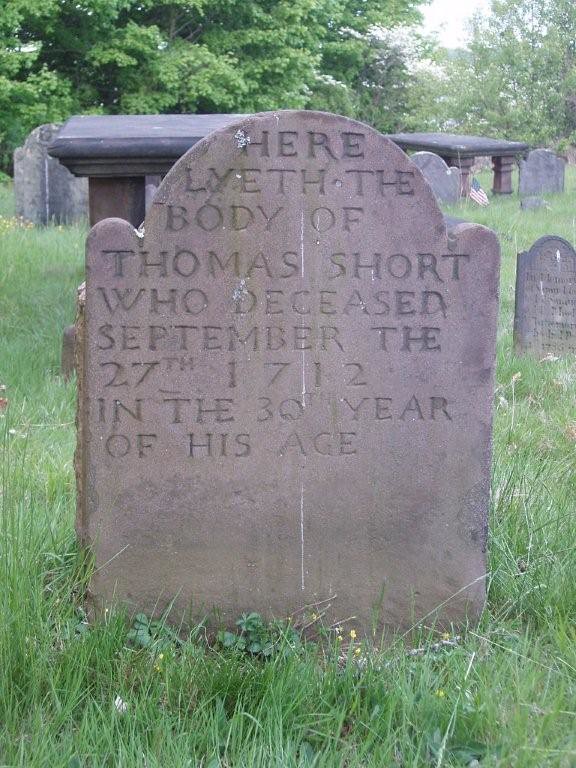In this tall, rectangular image of a graveyard, the central focus is an old, brownish-red tombstone. This headstone, which stands amidst very long grass, features a unique shape with a curved semicircle at the top flanked by two smaller semicircles, followed by a straight descent. The weathered stone, engraved at the top in all capital letters, reads: "HERE LIETH THE BODY OF THOMAS SHORT, WHO DECEASED SEPTEMBER THE 27TH, 1712, IN THE 30TH YEAR OF HIS AGE." Behind the tombstone, there is a larger, table-like tomb supported by legs, indicating another grave. To the right, distant among the tall grasses, and to the left, other similarly shaped old tombstones can be seen, contributing to the cemetery's historic atmosphere. In the background and along the horizon, several very tall, bright green trees stand tall against an overcast white sky, suggesting it might be the middle of a sunny day. Benches are also present in the cemetery, though further back. Overall, the image conveys a serene, yet solemn scene from a historic graveyard.